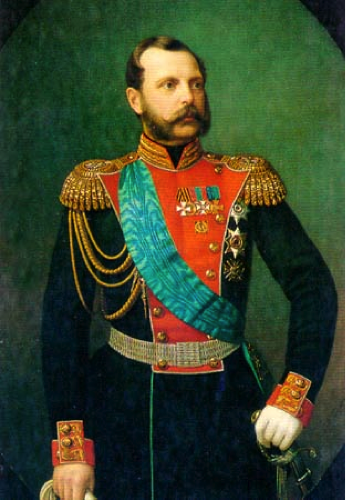The image is a historical painting of a European military figure from the 1800s, depicted as a white man with brown hair, a receding hairline, and large sideburns that extend to his chin. He also sports a mustache with curled ends. The background is a gradient from green to dark green, fading towards the bottom left corner. The man is portrayed facing forward but slightly turned to his left, looking in that direction. He is adorned in an elaborate navy blue or black military uniform with distinct red and gold embellishments. The coat features orange and red cuffs with gold buttons and intricate embroidery at the sleeves. Prominent gold epaulets adorn his shoulders, alongside gold fringes and cordage. A red section runs down the left side of his chest, adorned with various medals. Additionally, a striking blue sash with a possible tie-dye effect crosses his chest, complemented by a silvery metallic gold belt. In his left hand, he rests a gloved hand on the top of a sword's handle, while his right hand holds the accompanying white glove.